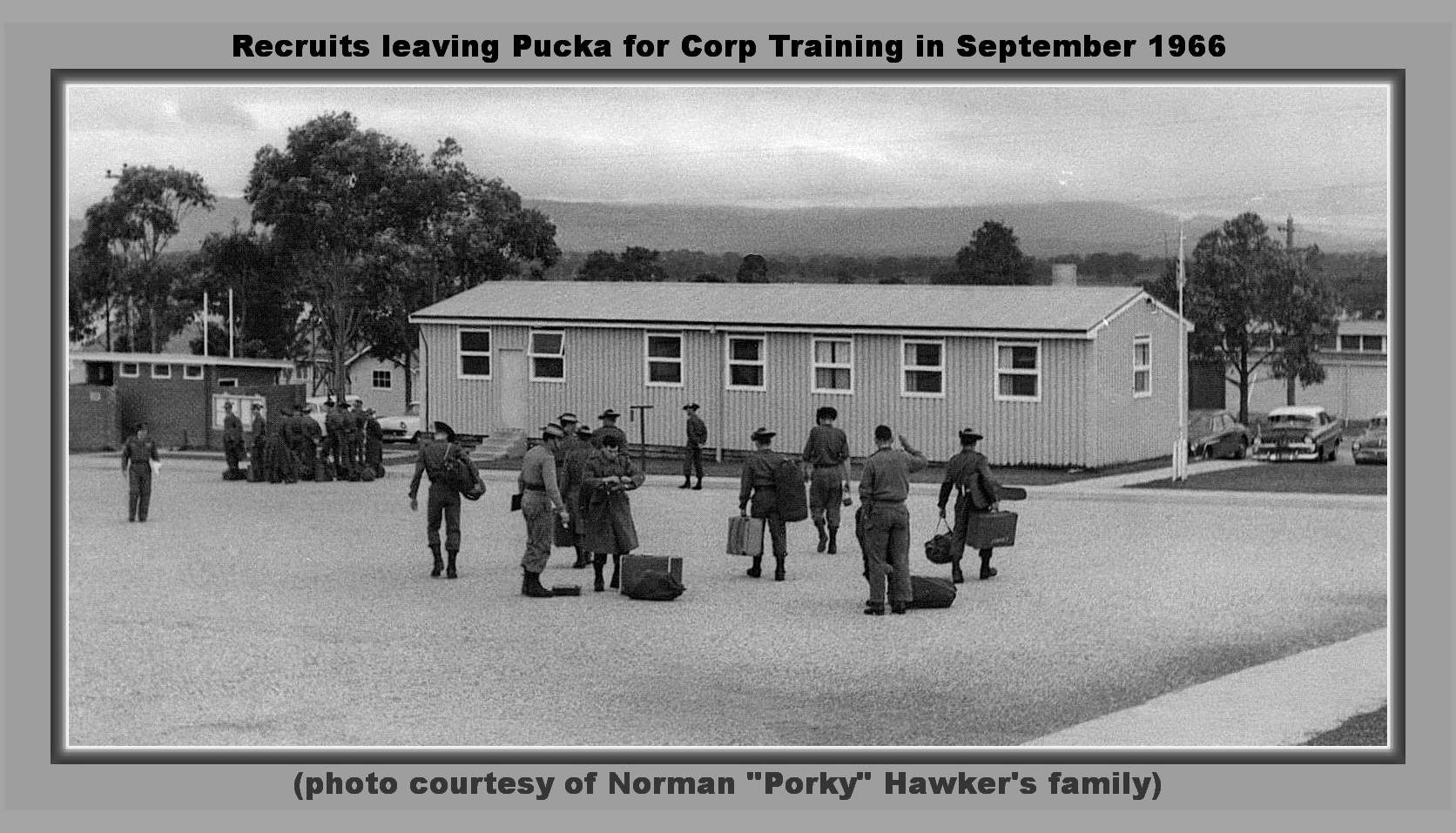This meticulously detailed black-and-white photograph, set against a gray rectangle background with a thin gray border and a thinner black border, captures a poignant moment from September 1966. At the top of the image, a caption in black font reads: "Recruits Leaving Pucca for Corps Training in September 1966." The scene showcases a lone, one-story barrack surrounded by a few houses. In the foreground, a wide, open field lays stretched out with men dressed in military fatigues, carrying their luggage, presumably heading towards their assigned training. The men appear poised on either a grassy field or perhaps some pavement. Beyond the barrack, a street is visible, lined with several old cars and additional houses. The background further extends into a not-so-high mountain range under a cloudy sky, enhancing the depth and mood of the moment. A note beneath the photograph states: "Photo Courtesy of Norman Porky Hawker's Family," adding a personal touch and historical authenticity to the image.